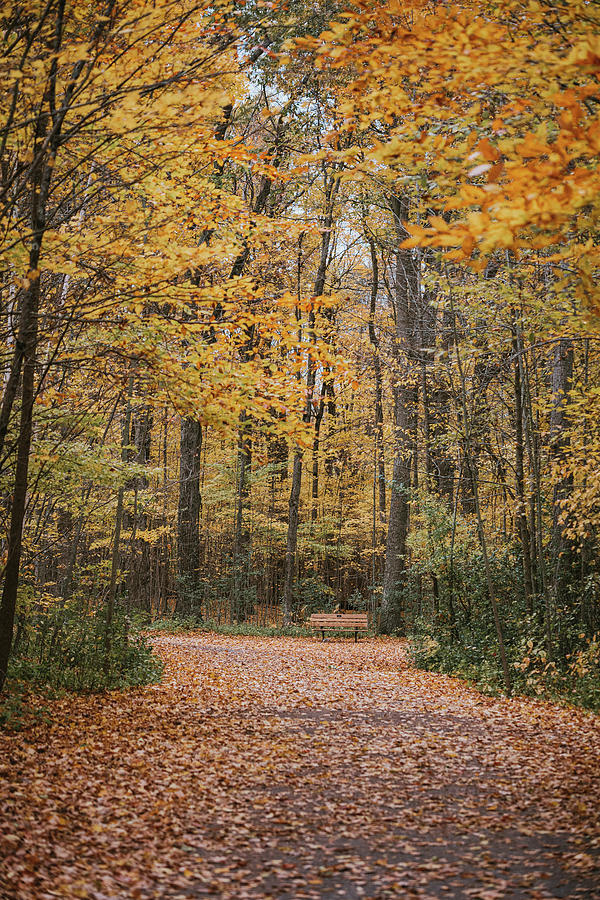A vibrant, peaceful autumn scene in a forested park portrays a well-paved, leaf-strewn pathway leading to a T-intersection, where a wooden bench sits unoccupied. The path and the area around it are blanketed in fallen leaves in rich hues of orange, yellow, and red, accented by green shrubs. Tall trees with gray trunks and dense foliage display a mix of yellow, orange, and green leaves, while a few bare branches signal the progress of fall. The blue sky peeks through the dense canopy, adding to the serene, daytime ambiance of this nature retreat.